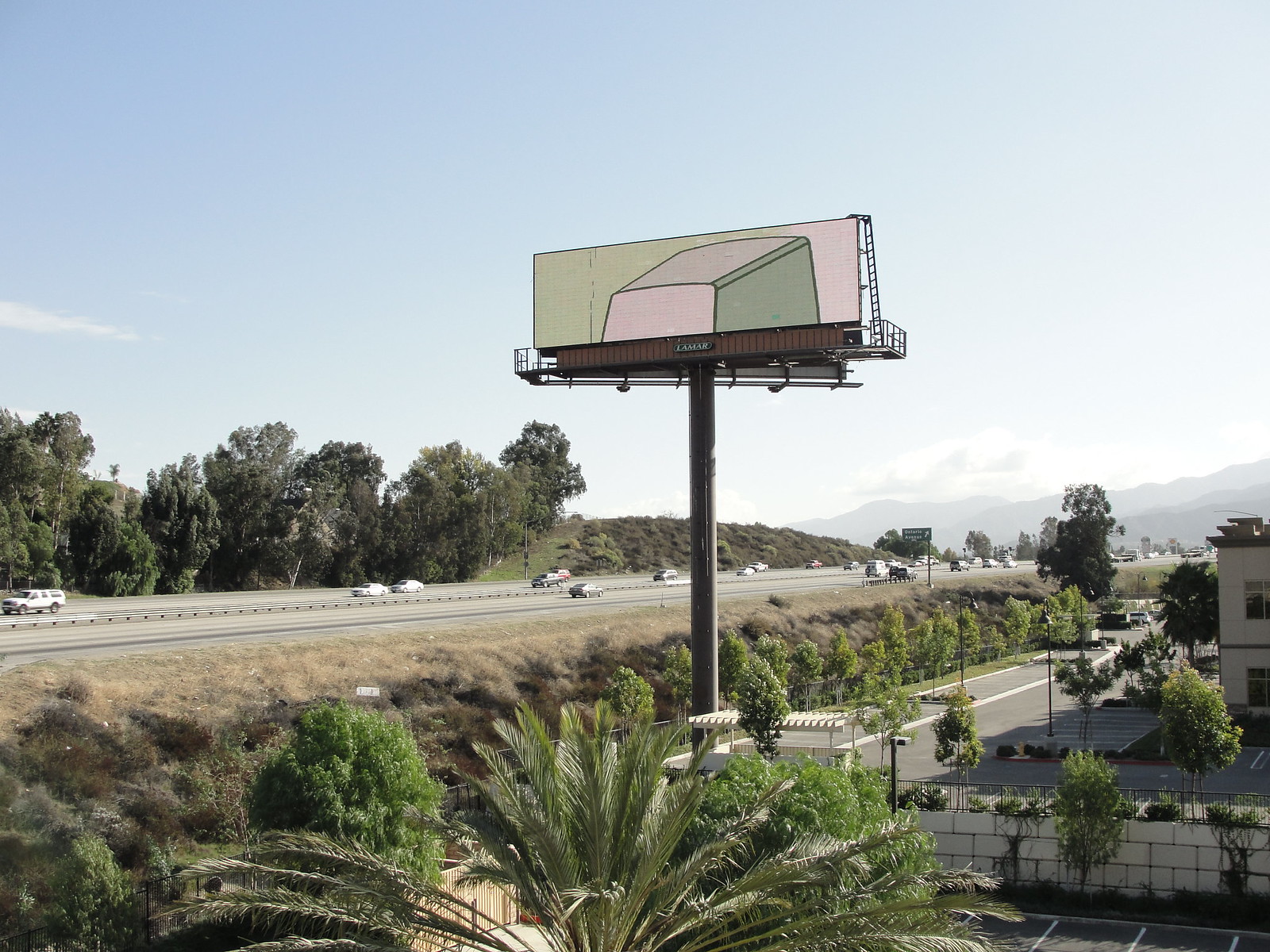In the foreground of this scene, a tall billboard stands on a thick brown metal pole, elevated by a scaffold. The billboard's background is divided into pale green and pale pink sections, and a 3D black ink outline renders the image of a box. The top and front sides of this drawn box are light pink, while one visible side is pale green; notably, there is no text on the billboard. Beneath the billboard, the ground features arid grass interspersed with bushes. To the side, a corporate building with a large parking lot is visible.

In the middle ground, an expansive highway stretches into the distance with vehicles traveling in both directions. Lining the far side of the highway are numerous large trees, beyond which lies a gentle hill.

The background is dominated by a distant mountain range under a bright blue sky dotted with a few white clouds. The picturesque scene is framed by green bushes with long, fanned-out leaves in the immediate foreground.